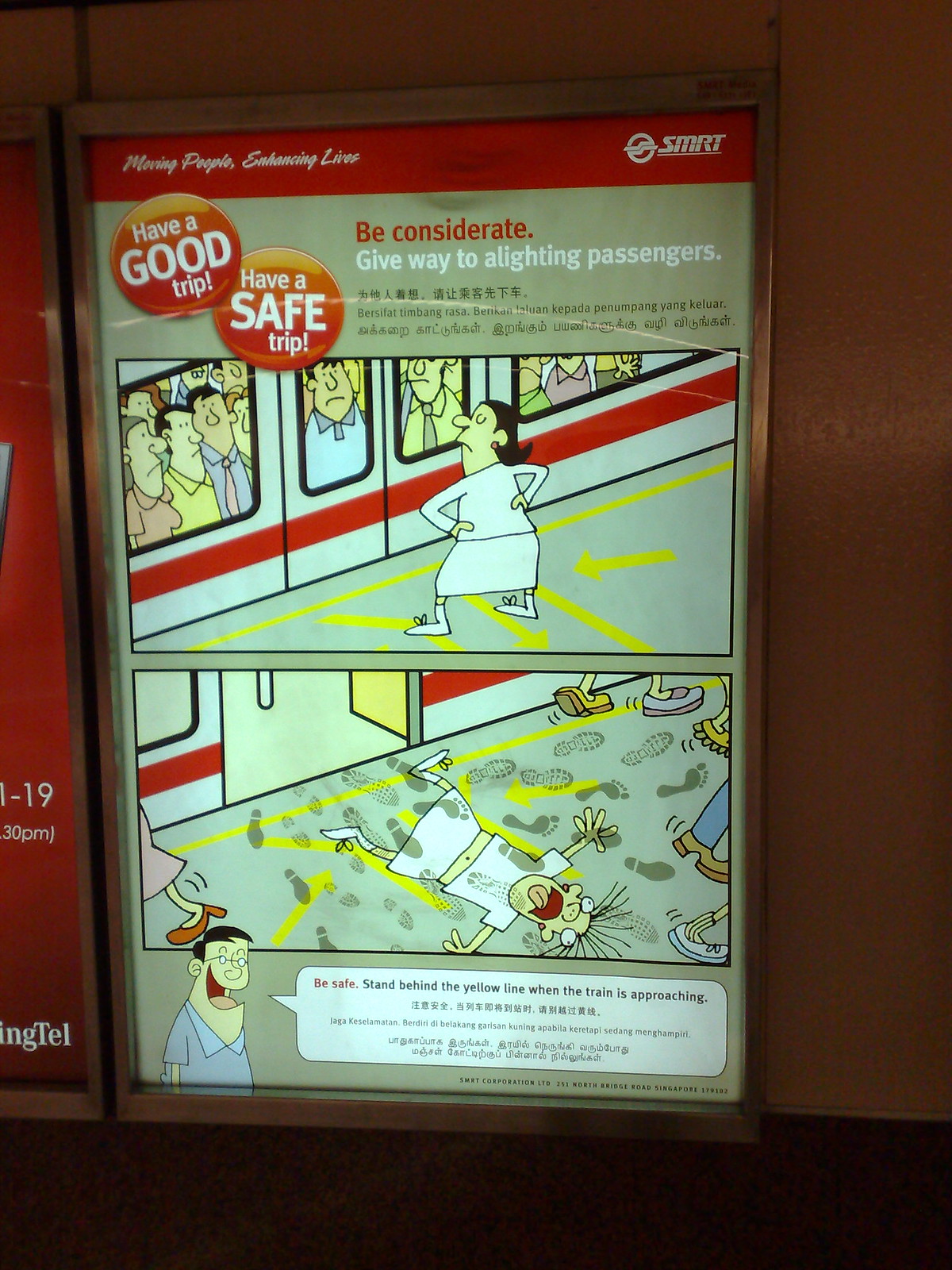This cartoon-style poster, mounted on a wall with a silver frame, appears to be part of a Rapid Transit or Transit Authority campaign. The top of the poster features a red border with the slogan "Moving People, Enhancing Lives," and to the right is a logo resembling an "S" with the letters "SMRT." A red icon reads, "Have a Good Trip, Have a Safe Trip." Below that, bold red letters say, "Be Considerate," followed by "Give Way to Alighting Passengers" in white text, accompanied by some Asian writing.

The poster is divided into two cartoon panels. The top panel illustrates a crowded train with passengers pressed up against the windows, while a frustrated woman with medium-length brown hair, dressed in a white long-sleeve shirt, skirt, and white shoes, stands on the platform beside the closed train doors with her hands on her hips. The train itself is gray with a horizontal red stripe.

The bottom panel reveals the aftermath: the train doors are open, and the same woman is sprawled out on the ground with footprints all over her, indicating that the passengers hurriedly exited the train, trampling her. The interior of the train is now empty. At the very bottom of the poster, an image of an Asian man wearing glasses is shown, reminding passengers to "Be Safe" and to stay behind the yellow line when the train is approaching.